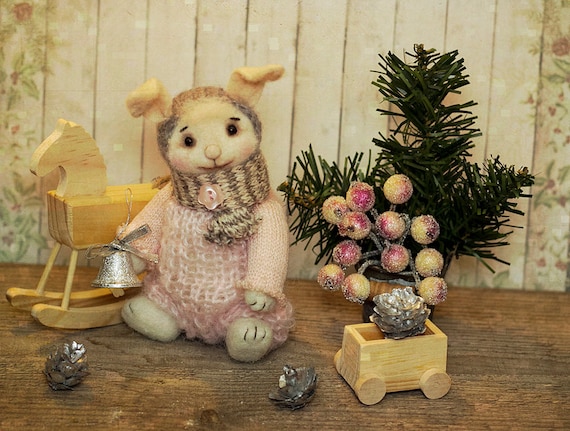The photograph portrays a charming, indoor scene featuring a white-painted wooden wall with visible dirt marks and painted leaves and plants on either side. In the foreground, a rustic wooden table or floor serves as the base for an assortment of toys and decorative items. A small wooden rocking horse is positioned to the left, angled towards the right. To the right of the horse, there's an adorable stuffed rabbit with floppy ears, dressed in a pink outfit, complemented by a scarf with a button fastening. The rabbit holds a small silver bell, adding a touch of whimsy to its detailed attire. Next to the rabbit, a wooden car holds a metal pine cone, with additional metal pine cones scattered on the table. Behind the car, a pine bush adorned with red and yellow berries adds a splash of natural color. The overall composition is warm and inviting, evoking a nostalgic, cozy atmosphere with a blend of light pink, fuchsia, dark green, grey, silver, and various wood tones.